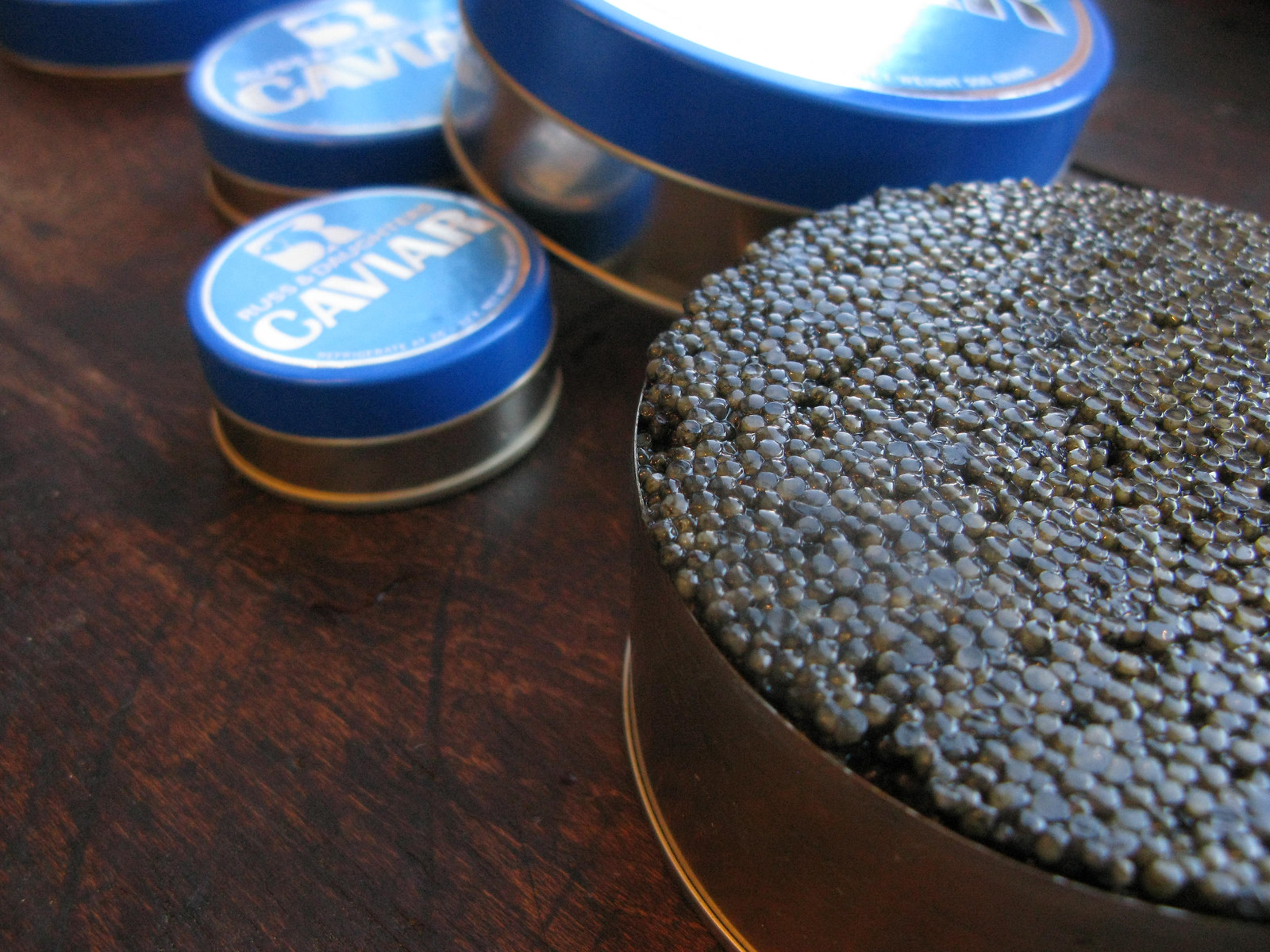This detailed photograph captures an assortment of caviar containers artfully arranged on a dark wooden table, characterized by subtle blackish striations and a slightly worn appearance. The focal point is a large round copper-colored tin in the right foreground, with its lid removed to reveal the glistening black pearls of caviar inside, their flat tops indicating the pressure exerted by the lid. Behind it, a similarly copper-bottomed, blue-lidded tin leans diagonally, slightly ajar, supported by two smaller, identical tins also featuring blue lids with white circles. These lids bear the inscription "Russ & Daughters Caviar," though the text is somewhat blurred. Additionally, there are two larger tins aligned with these smaller containers, contributing to the diverse yet harmonious arrangement of the caviar tins on the richly textured table.